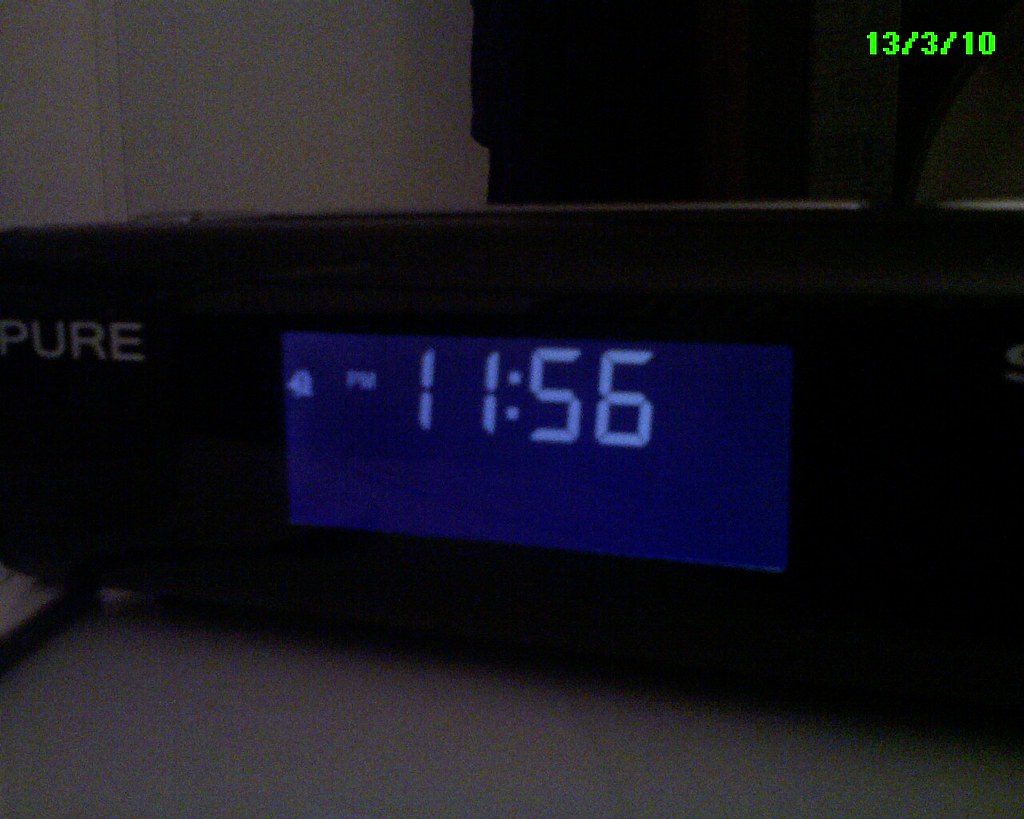The image is a close-up shot of a modern alarm clock, situated on a white bedside table against a white wall. The clock has a black frame with a blue LED display, showing the time as 11:56 PM in light blue or whitish digits. The brand name "PURE" is visible on the left side of the clock. A small alarm bell icon is present on the display, indicating an active alarm. In the upper right corner of the image, the date is displayed in neon green, reading 13/3/10, suggesting the photograph was taken on March 13, 2010. The background also features some indistinct code or text on the wall.